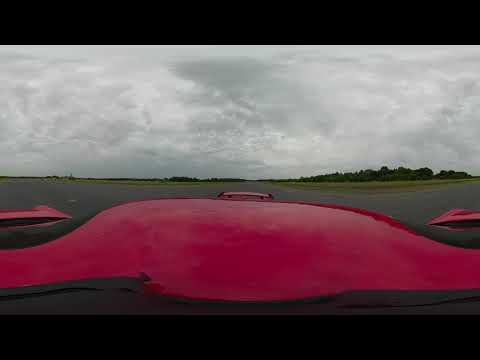The image captures an outdoor scene on a very overcast, gray day with dark clouds covering the sky. The perspective is from a camera positioned on the roof of a red car, showcasing its glossy, red surface, a curved top, and sharp edges on the left and right sides, with a slightly arched spoiler at the back. The photo includes a black dashboard seen from inside the vehicle, surrounded by a black lining. The road in front of the car extends in three directions—left, straight, and right—covered with grey tarmac. Patches of green grass border the track, and a tree line runs horizontally across the background.